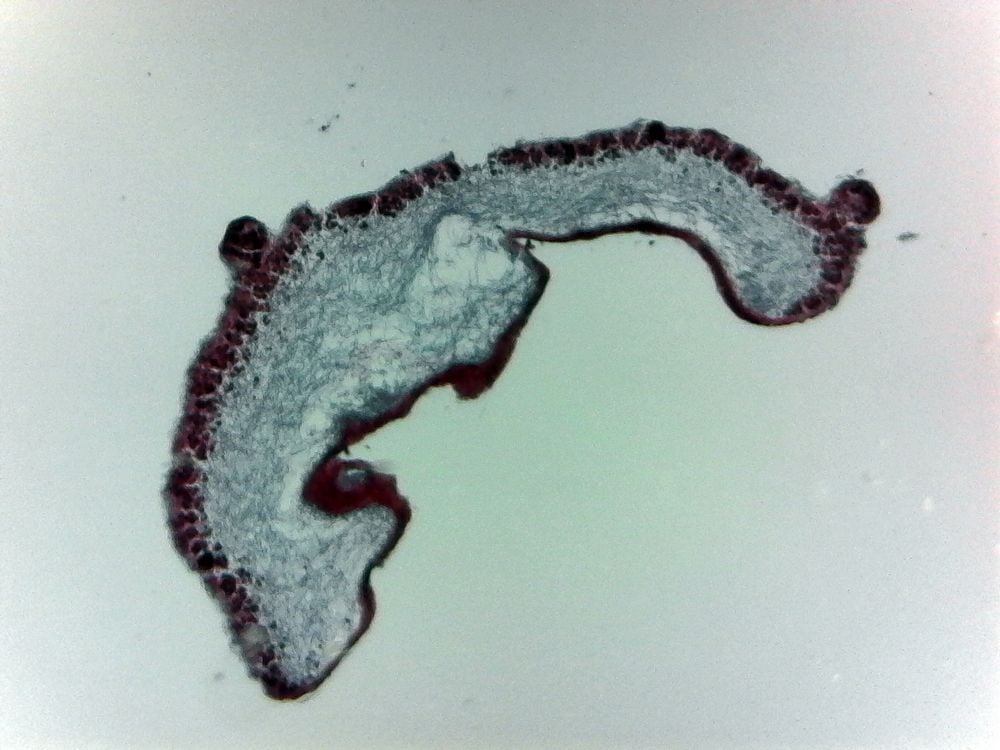The image under the microscope reveals a highly detailed scene set against a predominantly aqua-colored background, which fades to nearly white at the corners. The far left and right sides exhibit a slight pinkish hue, suggesting an aged or lower-quality image. Dominating the center is an organic, possibly aquatic organism or object, characterized by a thick, dark, potentially black outline. Notably, there are nodal extensions at the far right, top right, and top left of this central form. The outline encloses a web-like or materialistic interior with shades of black and light gray, resembling a stretched, elongated shape akin to a fish or seahorse. This interior structure includes a spine-like line with bubble-like nodes, possibly indicating anatomical features. The overall composition sits atop a backdrop that shifts between pale blue and white, creating a sense of depth and microscopic scrutiny.